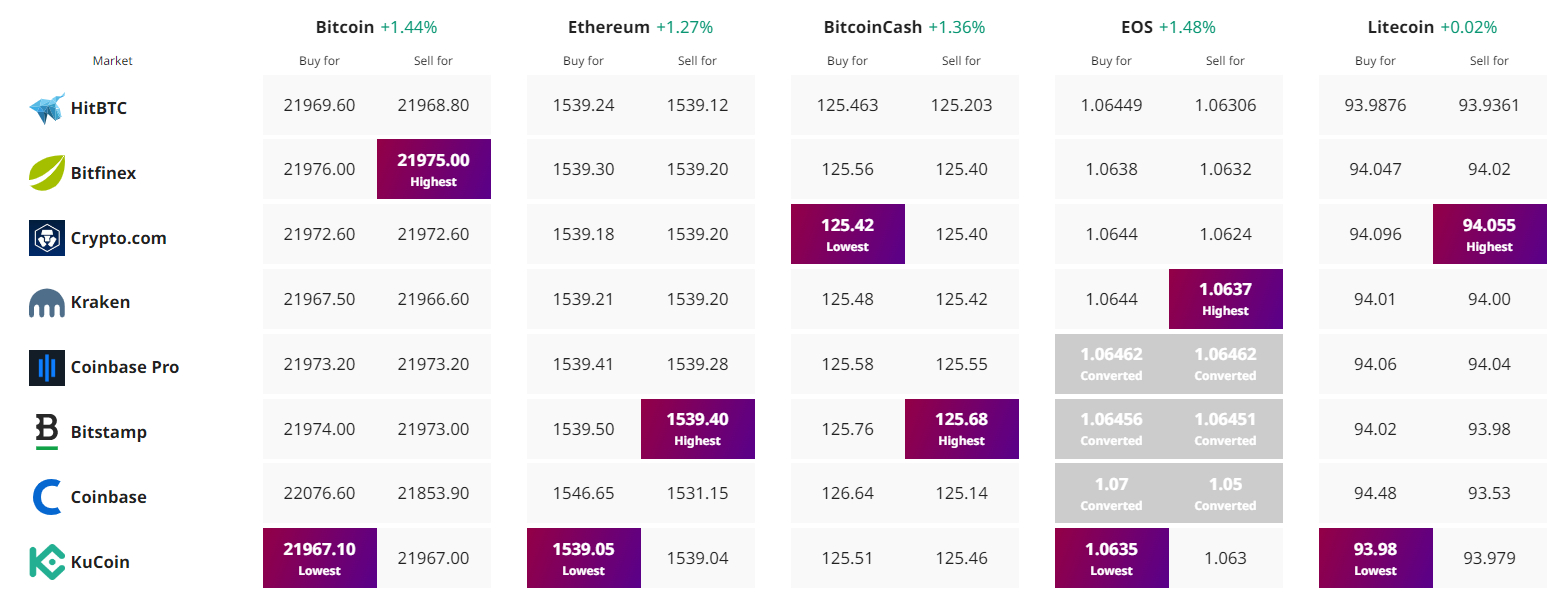The image depicts an online cryptocurrency trading platform, featuring a bidding page. At the very top, the page is labeled "Market". Below this heading, several well-known cryptocurrency exchanges are listed with their respective logos, including Crypto.com, Kraken, Bitfinex, Coinbase, and KuCoin. Each exchange is presented in its own segment, predominantly using colors like gray and purple. For each listed exchange, there are options clearly marked as "Buy For" and "Sell For", where these actions are highlighted in purple boxes. The overall theme of the page includes a mix of gray and plum-colored elements, creating a structured yet colorful interface dedicated to trading cryptocurrencies.